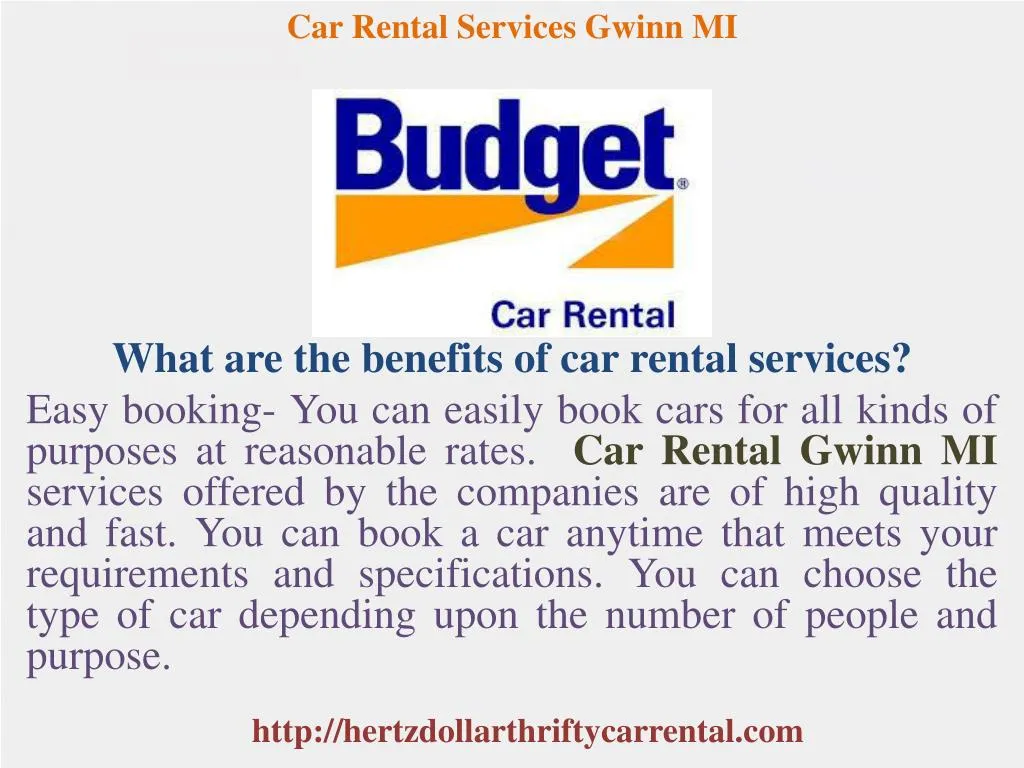The image features a promotional poster for a car rental service, primarily highlighting Budget Car Rental. The background of the poster is a light gray color, providing a subtle and neutral foundation. In the top center of the poster, the text "Car Rental Services G, win, M, I" is displayed in a sophisticated gold-colored font, lending an elegant touch to the design.

Centrally positioned beneath this text is a prominent white rectangular box. At the top of this box, the word "Budget" is written in a large, bold blue font, making it the focal point of the poster. Directly below "Budget," a gold bar is placed, starting thick on the left and progressively tapering to the right, adding a sleek visual element. In the bottom right corner of this white box, the term "car rental" is included in a smaller font.

Further down the poster, outside the white box, a title is presented in a darker blue font that reads, "What are the benefits of car rental services?" Following this title, a paragraph in a lighter purple font begins with the phrase "easy booking," hinting at the convenience offered by the service. Finally, at the bottom of the poster, the web address "HertzDollarThriftyCarRentals.com" is provided, directing potential customers to their online platform.